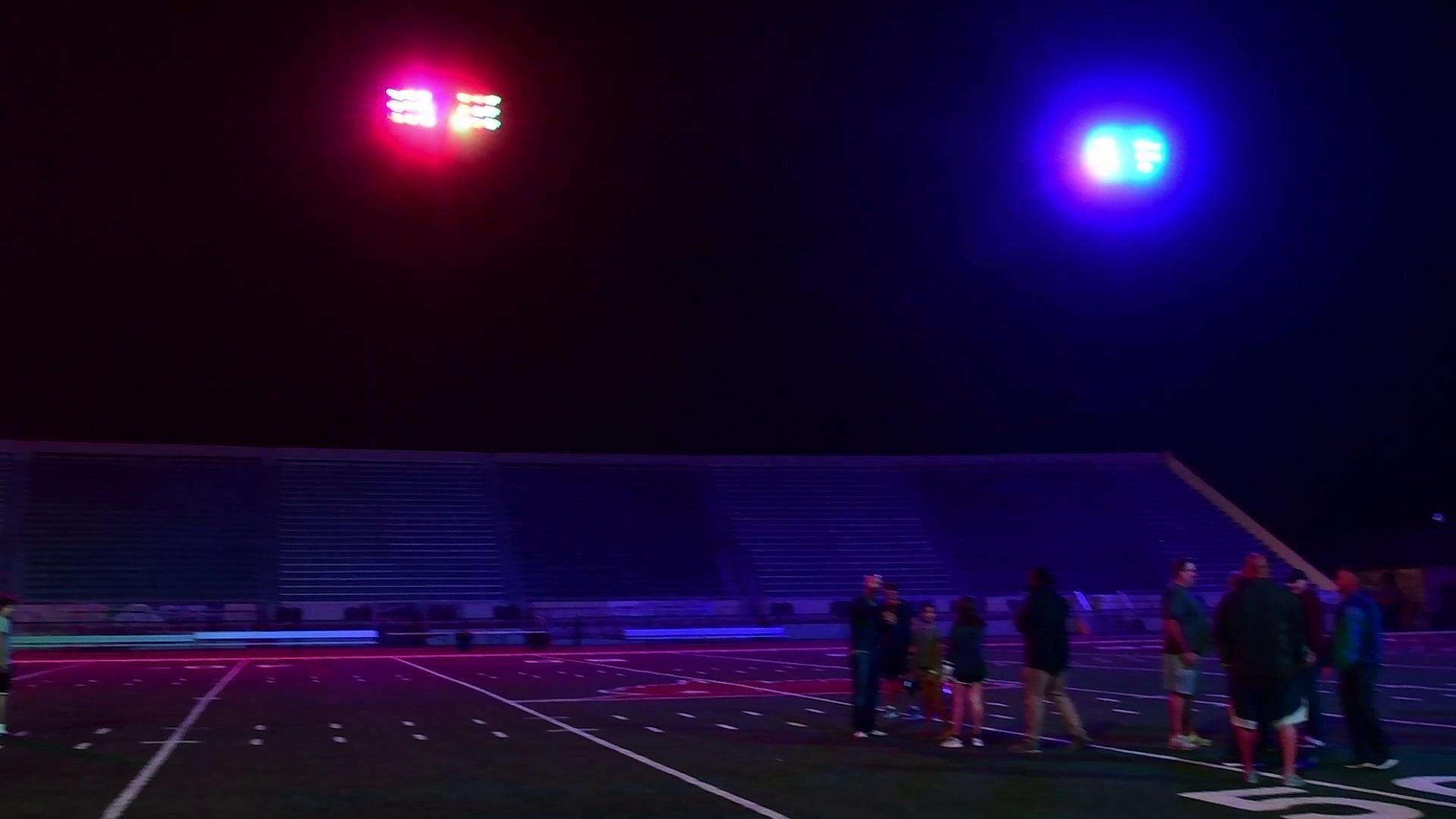The photo depicts a small American football field at night, reminiscent of those found in high schools or small universities. The field is illuminated by distinctive red and blue lights, with the reds to the left and blues to the right, both mounted high on poles over the bleachers. These lights cast colorful hues across the field and onto the forward part of the stands.

In the foreground, there are two groups of people gathered on what appears to be the 50-yard line. The group on the right consists of several men standing in a circle, engaged in conversation. Close by, another group includes a woman, a man, and a few children, also huddled together. The bleachers in the background are completely empty, with no ongoing game or players on the field, suggesting it might be a practice session or an off-time during summer, as some people are dressed in short pants. The serene and somewhat eerie ambiance is highlighted by the stark contrast between the vibrant lights and the dark night sky.